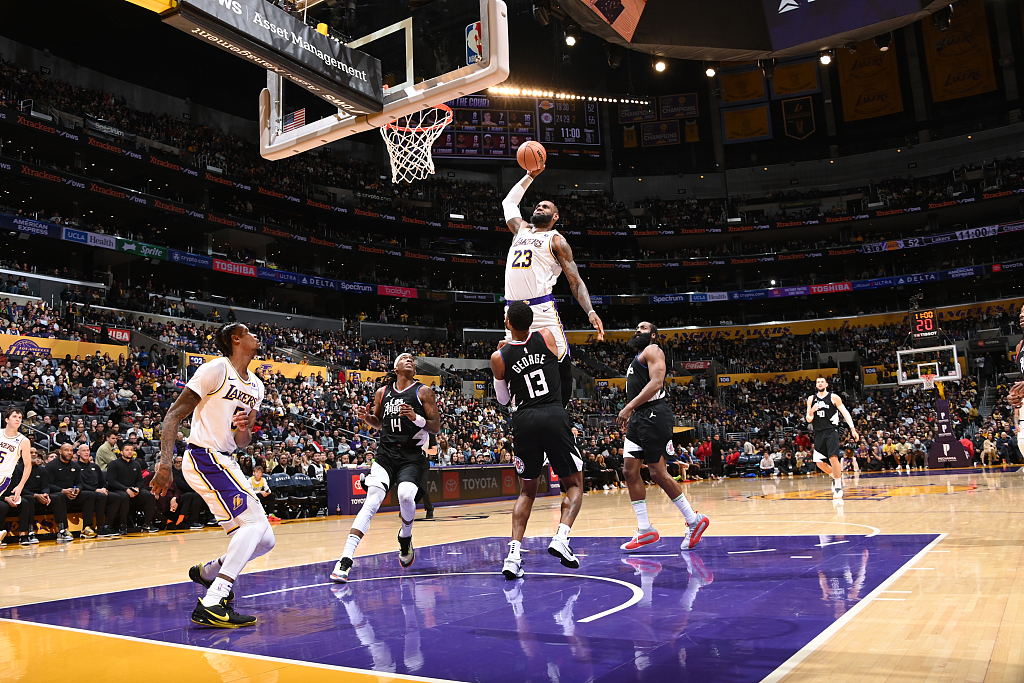In this dynamic photograph of a high-stakes basketball game between the Los Angeles Lakers and an opposing team in black uniforms, LeBron James, wearing the Lakers' white uniform with purple and yellow accents, is captured mid-air with the basketball in hand, poised to execute a powerful slam dunk. The scene is set against the vibrant backdrop of a packed Lakers stadium, with thousands of spectators intently watching the action unfold on a court colored in gold, purple, and beige. LeBron, sporting jersey number 23, is surrounded by teammates and opponents alike, including a player wearing a black jersey with "George, 13" emblazoned on it. The intense concentration on LeBron's face and the collective anticipation of the audience highlight the electrifying atmosphere of this pivotal moment in the game.